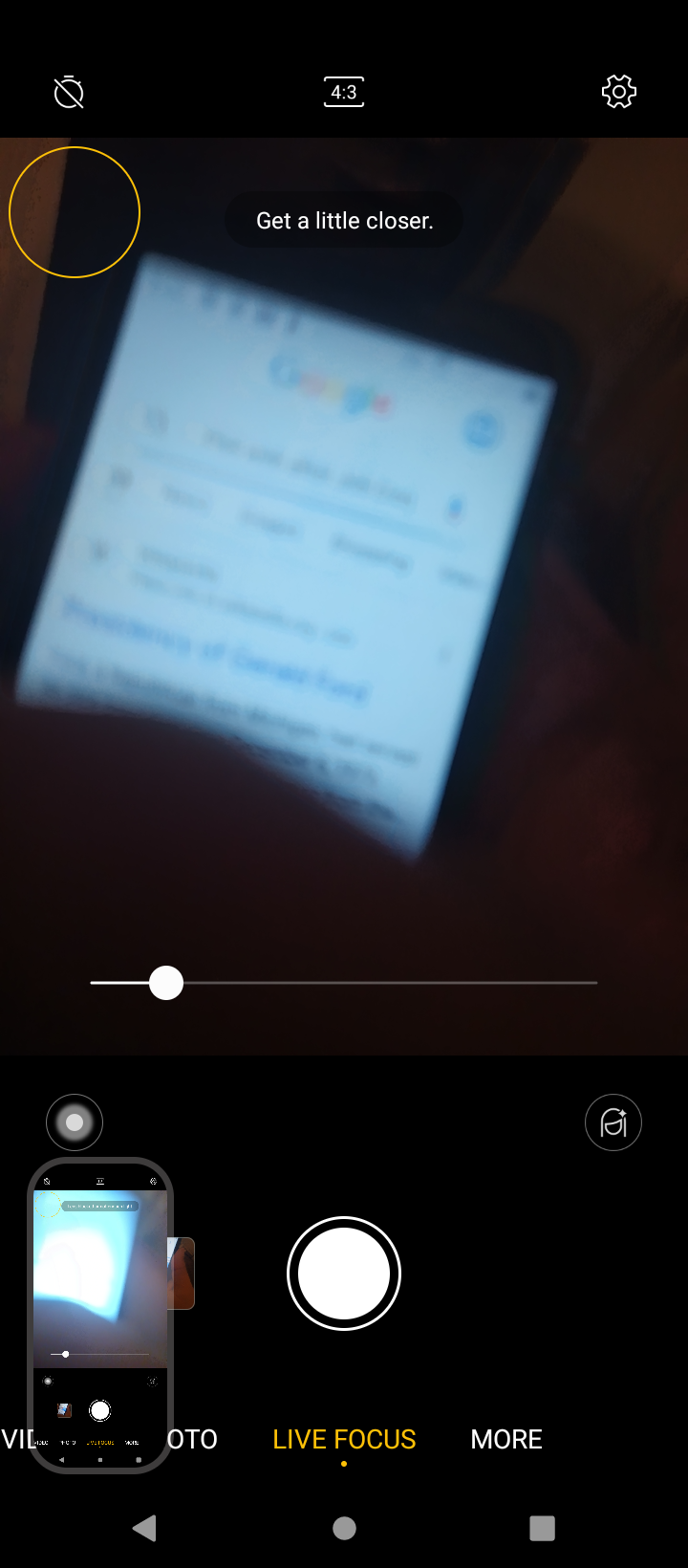In the image, we observe a live focus screenshot taken from a cell phone capturing another device displaying the Google homepage. The photograph is vertically rectangular, representing the cell phone's face which holds the image. The background is predominantly black with the icons for settings, including a gear symbol, shown at the top. The notification bar also contains an orange circular icon along with a "4:3" ratio display. The screen of the second device is lit, presenting a Google search page with the Google logo prominently featuring the letters "G" in blue, "o" in red, "o" in yellow, "g" in blue, "l" in green, and "e" in red against the white background, though the search query remains indistinct and out of focus. Displayed centrally in white text, the screen prompts, "Get a little closer." 

Directly below this, a light bar with a white dot and thin white line is visible, followed by a white circle with a black outline and a thin white circular border. Toward the image's base, an orange caption reading "LIVE FOCUS" is centrally placed, while the word "MORE" appears in white on the right. The screen also contains a version of the image overlaid in the lower left corner. The bottom ribbon houses the camera interface with a backwards button, a central circle button for taking the picture, and a square button, all in light gray.